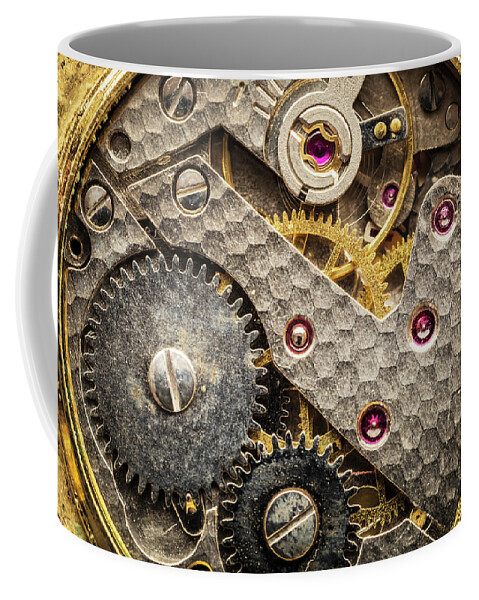This is a high-resolution photograph featuring a close-up view of a uniquely designed mug set against a pristine white background. The mug's interior and handle are immaculately white, with the handle subtly visible on the left side of the image. The exterior of the mug is adorned with an intricate and detailed painting that showcases an assemblage of interlocking gears and metal components. These gears are beautifully rendered in a rich palette of silver, gold, and bright purple hues, with bolts of matching colors—some in glittering silver and others in vibrant purple—enhancing the mechanical motif. The craftsmanship and attention to detail in the painted design make this mug a striking fusion of art and utility.